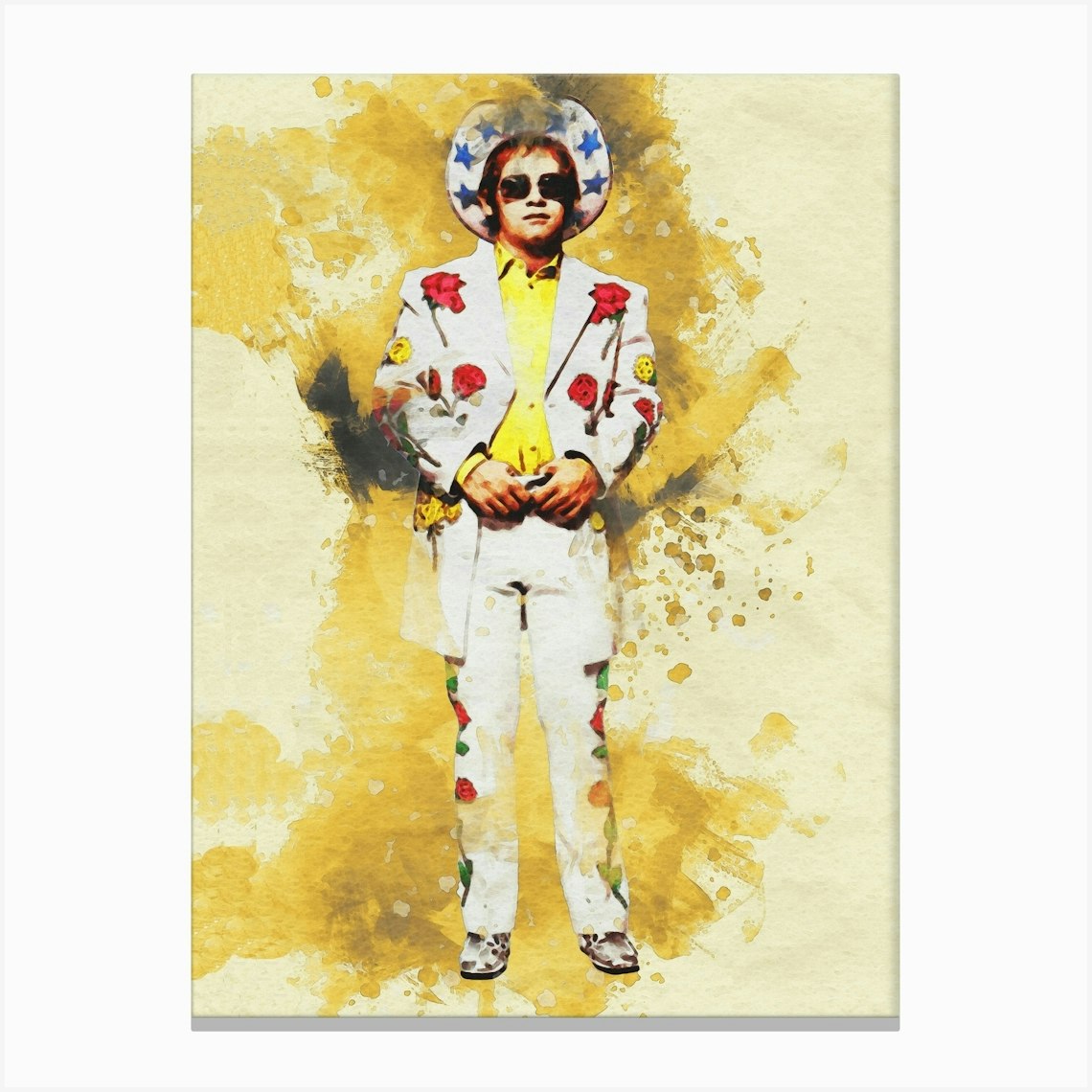The painting depicts the iconic rock singer Elton John in a vividly detailed, realistic style, set against a solid white background typical of commercial product photography meant to direct focus entirely on the artwork. The rectangular poster features a light yellow base with dark yellow and black splotches behind Elton John, enhancing the visual appeal. Elton John is dressed in an eye-catching white cowboy suit adorned with red roses on his shoulders and down the sides of his legs, yellow flowers on the back of his jacket sleeves, and additional orange flowers on his forearms. His ensemble includes silver cowboy boots and a prominently tilted white cowboy hat with blue stars around the rim. He is also wearing dark square sunglasses and a yellow button-down collared shirt under his jacket. Elton John stands gripping his belt buckle with both hands, an expression of youthful confidence highlighted by his brown hair glimpsed under the hat. The meticulous detail in the painting captures the essence of a younger Elton John, making it a remarkable depiction of the legendary musician.